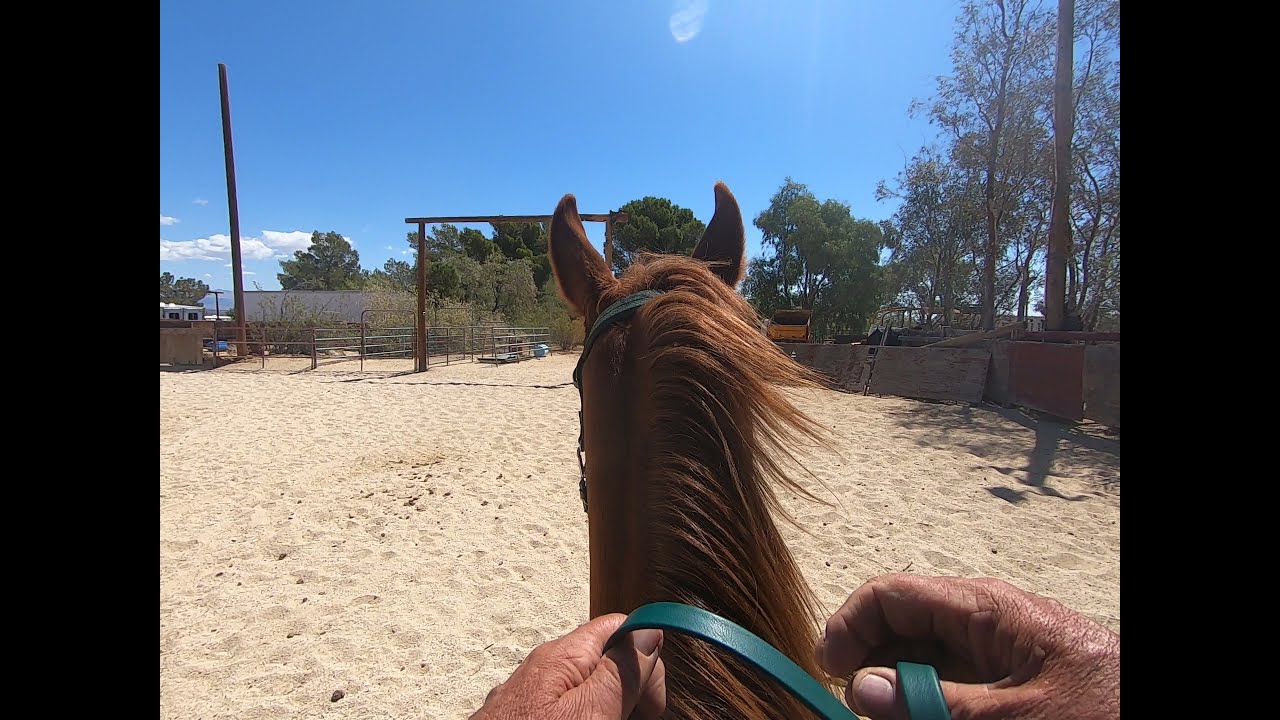This outdoor photograph captures the thrilling, first-person perspective of a person riding a brown horse with long neck hair and prominent ears. The image seems to be shot from chest level, showing the rider’s slightly dirty hands gripping a blue harness as they navigate a sandy, cream-colored terrain scattered with footprints. Surrounding this sandy area is a sturdy boundary made of bricks and metallic fences, with a visible gateway for entry and exit. Beyond the enclosure, lush trees with verdant green leaves stretch out, under a clear blue sky adorned with a few scattered clouds.